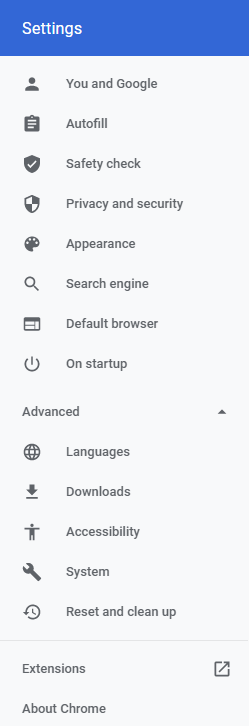The image showcases a screenshot of Google Chrome’s settings menu, depicted with a blue bar at the top. On the left, "Settings" is prominently displayed in white. Below this, a series of gray icons and their corresponding labels are listed sequentially:

1. A small person icon with the label "Google India".
2. A clipboard icon marked "Autofill".
3. A checkmark icon indicating "Safety Check".
4. A shield icon denoting "Privacy and Security".
5. An art easel icon for "Appearance".
6. A magnifying glass icon labeled "Search Engine".
7. A small browser icon indicating "Default Browser".
8. A power symbol labeled "Startup".
9. An "Advanced" section with an arrow pointing up on the right side.
10. A globe icon for "Languages".
11. A down arrow underlined labeled "Downloads".
12. An icon of a person performing a dance gesture labeled "Accessibility".
13. A wrench icon indicating "System".
14. A clock with a circular arrow labeled "Reset and Clean Up".
15. At the bottom, an option marked "Extensions", represented by a square with an arrow pointing to its upper right corner.
16. The final item is labeled "About Chrome".

Each icon is meticulously paired with its function, providing a comprehensive overview of the settings menu.